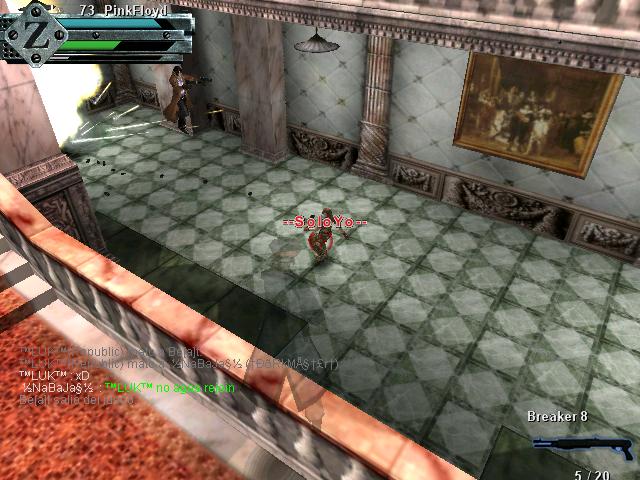Screenshot from a third-person shooter multiplayer video game. The user interface (UI) displays a chat log in the bottom left-hand corner, indicating active communication with other players. In the upper left-hand corner, a sleek, metallic-designed UI element shows health bars with blue and green indicators, though their specific meanings are unclear. The text "73 Pink Floyd" is printed above the health bars. In the bottom right corner, an image of a shotgun is displayed, labeled "Breaker 8" with an ammunition count of "5/20." 

The scene captures two characters, one levitating in the air dressed in brown and blue, and another on the ground labeled "Solo Yo" in red. The environment features a green and white tiled floor, white walls with tan-colored pillars, a faux stone artifact hanging on the wall, and a brown-colored painting, creating a richly detailed and immersive setting.